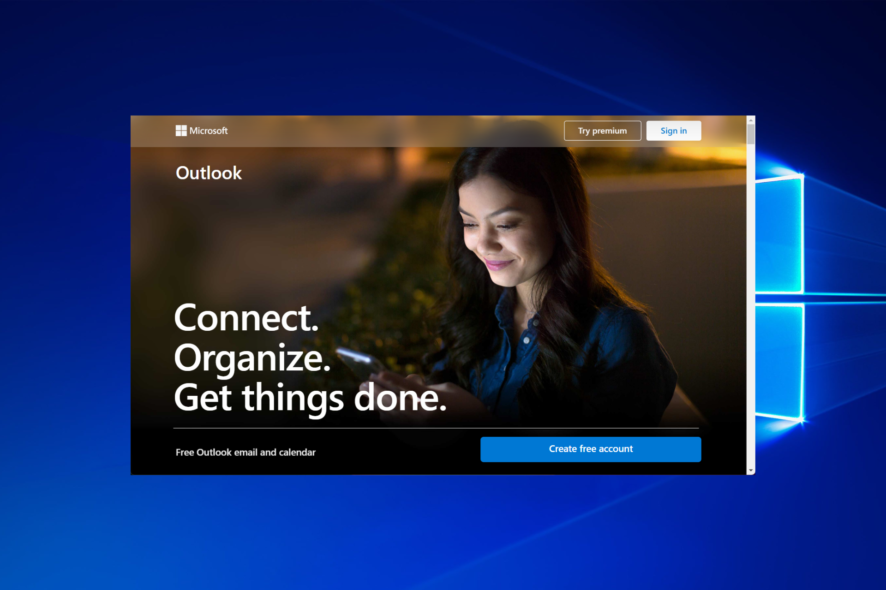The computer screen displays a vibrant advertisement for Microsoft Outlook, which features a smiling woman engrossed in her cell phone. The ad emphasizes key benefits of Outlook with the phrases: "Connect, organize, get things done." Below these slogans, the text invites users to "Create free account for free Outlook email and calendar." At the top of the screen, there are options to "Try premium" and "Sign in," suggesting access to enhanced features and existing accounts. This setup screen, likely part of the initial setup process for a new computer, sits against a striking blue background emblazoned with the brightly lit Windows logo, composed of a series of cubes mimicking window panes. The advertisement appears to be floating in the center of the screen, clearly showcasing the pre-installed software that accompanies new Windows devices.